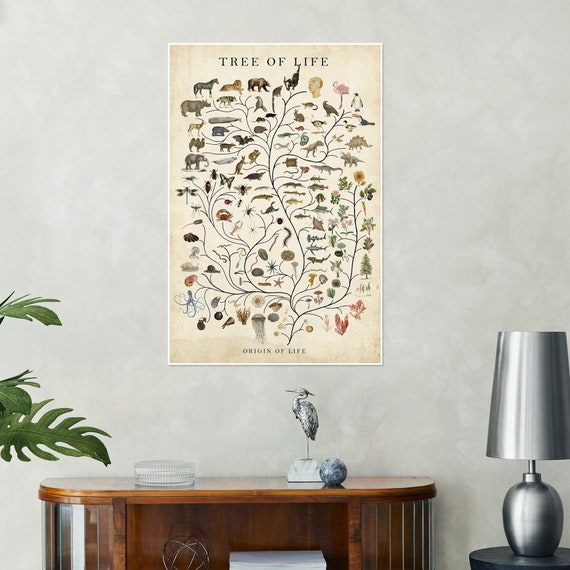In a serene room adorned with grey walls, a remarkable artwork titled "Tree of Life" dominates the scene. The intricate picture showcases a tree with many tiny branches, teeming with various animals like horses, lions, bears, and birds, interspersed with vibrant yellow and red flowers and green foliage. At the bottom of the artwork, the phrase "Origin of Life" is inscribed, encapsulating the essence of the piece. Below this captivating artwork stands a dark cherry wood desk, topped with a striking silver bird statue and a ceramic ball, adding an artistic touch. To the right of the desk, a small black table holds a sleek, metallic lamp, contributing to the room's elegant and harmonious aesthetic.